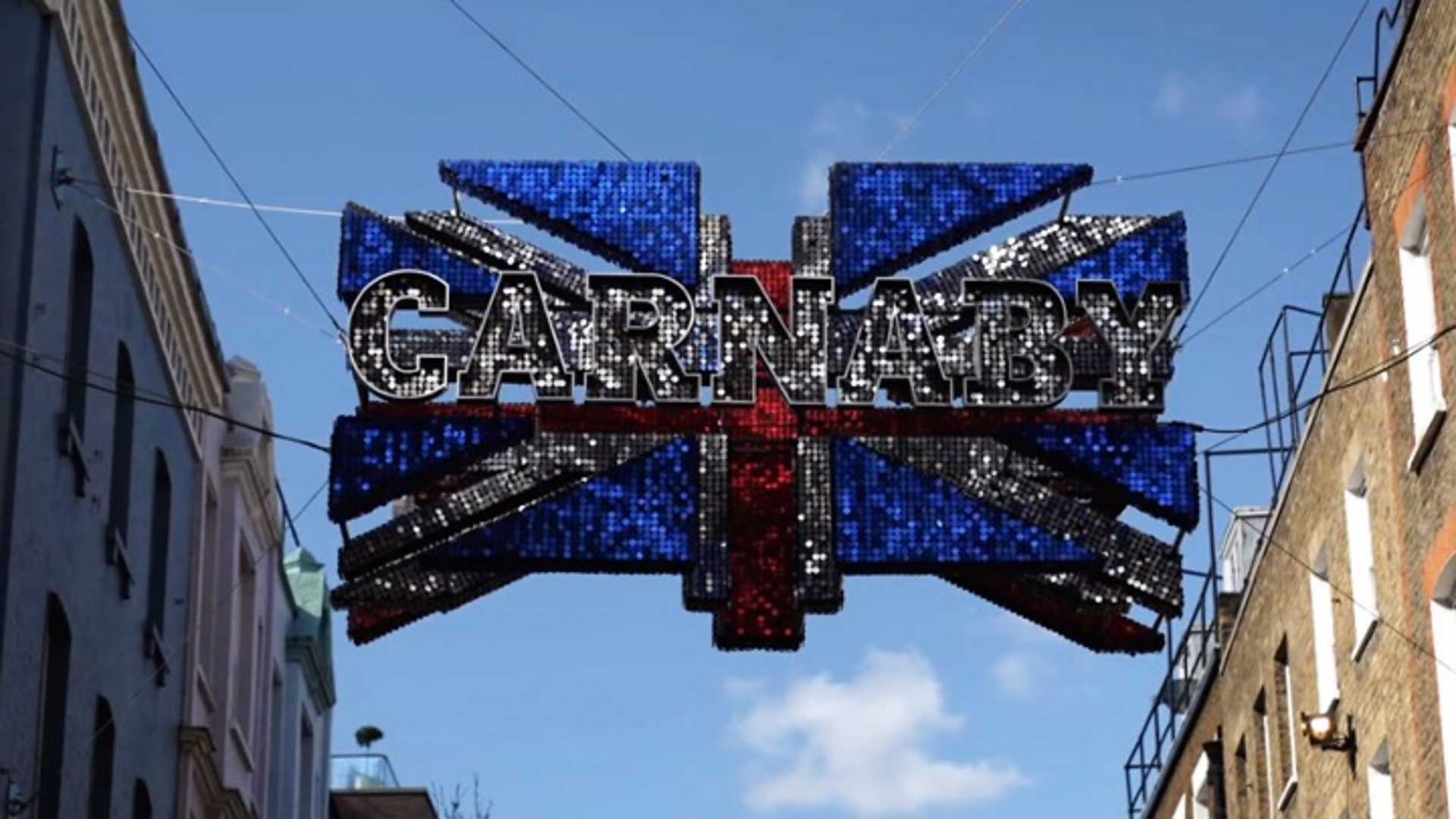This photograph, taken from below on a sunny day, captures a vibrant, outdoor city scene. Dominating the image is a large, glittering banner that stretches between rows of buildings, almost forming an arch over the unseen street below. The banner, securely strung by ropes attached to the buildings, proudly displays the word "Carnaby" in big, silver, shiny block capital letters. Behind these letters is a three-dimensional design of the British flag, rendered in a mosaic of blue, red, and silver colors, augmented by sequins and LED lights. 

The buildings flanking the banner add to the urban charm. The left side features structures with colored facades, primarily darker hues, including blue and black. Meanwhile, the right side is lined with tan and brown brick buildings. The bright, light blue sky, dotted with minimal fluffy white clouds, serves as a backdrop, enhancing the banner's glittering effect and contributing to the image's lively atmosphere. Numerous wires crisscross above, adding another layer of texture to this bustling city scene.